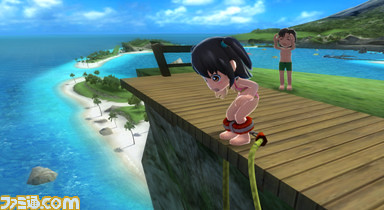In this vibrant and whimsical cartoon scene, inspired by a K-movie aesthetic, an expansive azure sky forms a breathtaking backdrop, adorned with a distant mountain that adds depth to the landscape. The setting is a picturesque coastal area, with the sprawling ocean meeting a lighter blue inlet, creating a serene transition in the water's hues. Beachy expanses stretch along the shore, and a natural sandy bridge delineates the inlet from the open ocean. Dominating the foreground, a rugged cliff is topped with a wooden boardwalk, from which two animated characters embark on their adventure. A boy clad in a bathing suit stands to the side, while a girl, with bungee cords securely fastened around her ankles, crouches in anticipation, poised to leap into the exhilarating unknown below.